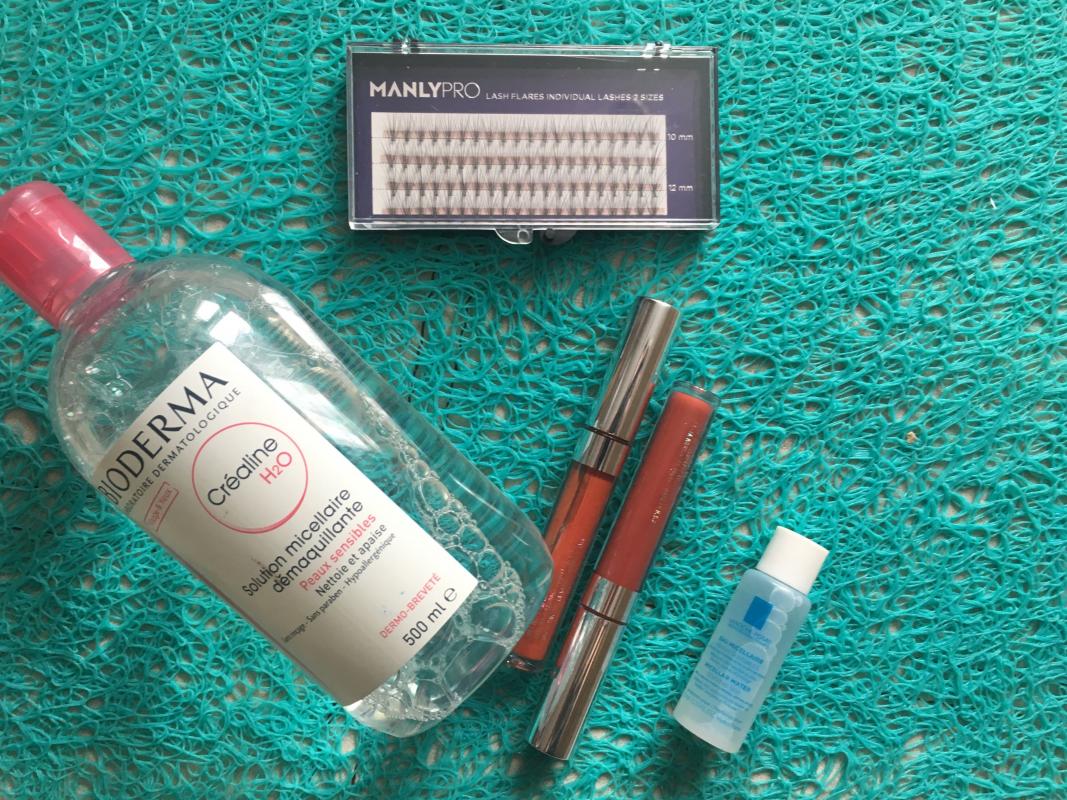On a light blue table covered with an aqua blue, net-like fabric dotted with small holes, a variety of beauty products are arranged. The centerpiece is a large, clear plastic bottle of Bioderma Crealine H2O, a renowned micellar water for skincare. The product label features the text "Bioderma Creoline H2O" with "H2O" highlighted in red within a red circle. The bottle also reads "Solution Micellaire Démaquillante," indicating its function as a makeup remover.

To the side, there's an orange-colored lipstick encased in clear plastic with a silver cap, alongside another lipstick in a more rosy hue, also featuring a silver tip. Additionally, a small white bottle with blue writing and a white cap is visible, containing a clear gel substance.

Moreover, a plastic box with a clear top and a black bottom rests prominently on the table. Inside, a black background sets off the white text "Manly Pro," identifying the product as individual fake eyelashes rather than a full lash set. This thorough display of beauty essentials is meticulously organized, offering a complete view of the various items.